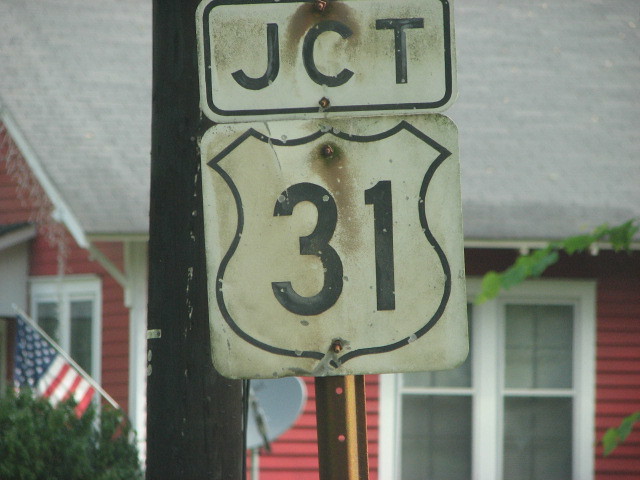In this vibrant daytime outdoor photo, the main focus is on a street sign prominently displayed in the foreground. The upper part of the sign features a rectangular pane with a black rim and rounded corners. Inside, in bold black capital letters, it reads "JCT." Below this, a square white sign with rounded corners is attached, displaying the number "31" inside a black-outlined shield shape. The background reveals a picturesque red-sided house with a gray peaked roof and white-trimmed windows. An American flag is proudly hung at the side of the house, where a satellite dish is also noticeable.